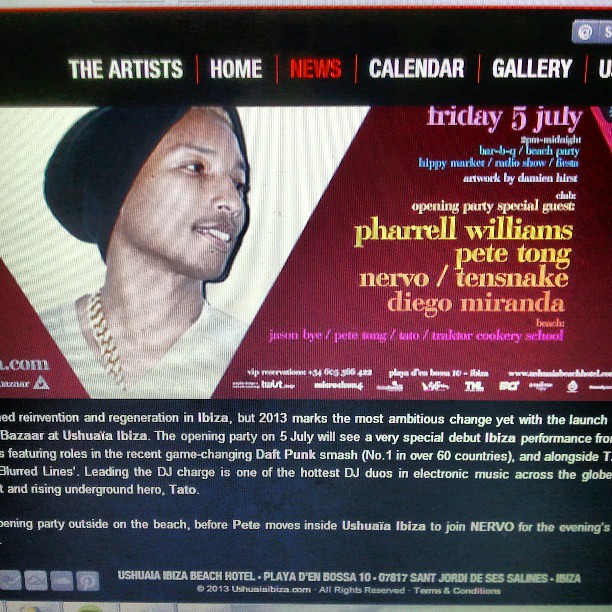The image depicts a website with a black navigation bar at the top, featuring tabs labeled "The Artist," "Home," "News," "Calendar," and "Gallery." The "News" tab is highlighted in red, indicating the current page, while the other tabs are white. The page details an event scheduled for Friday, July 5th, from 2 PM to midnight, highlighting a beach party barbecue with a hippie market, radio show, and fiesta. Special guests include Pharrell Williams, Pete Tong, Nervo, Tensnake, and Diego Miranda. 

To the left, there is an image of Pharrell Williams. Below the main event details, additional information about unrelated offers at the bazaar at Usala Ibiza is noted. Towards the bottom of the page, the website footer includes text reading "Ushah Baeza Beach Hotel" along with a copyright notice from 2013.